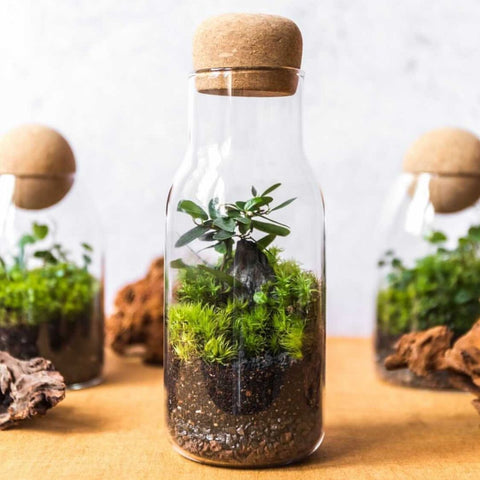The image displays several cylindrical glass vials, each topped with a rounded, wooden brown cork. Inside the vials, the bottom quarter to one-third is filled with brown soil, from which small green plants sprout, including tiny grasses and a distinct, darker green plant resembling a miniature tree. The vials are set on a light brown tabletop, surrounded by rocks in shades of pink and orange. In the background, more glass bottles can be seen, slightly different in shape and blurred to emphasize the central bottle. These background bottles similarly contain soil and diverse green plants, suggesting they are terrariums. The upper portion of the background is a mix of white and grey, further drawing focus to the detailed, vibrant greenery within the central vial.